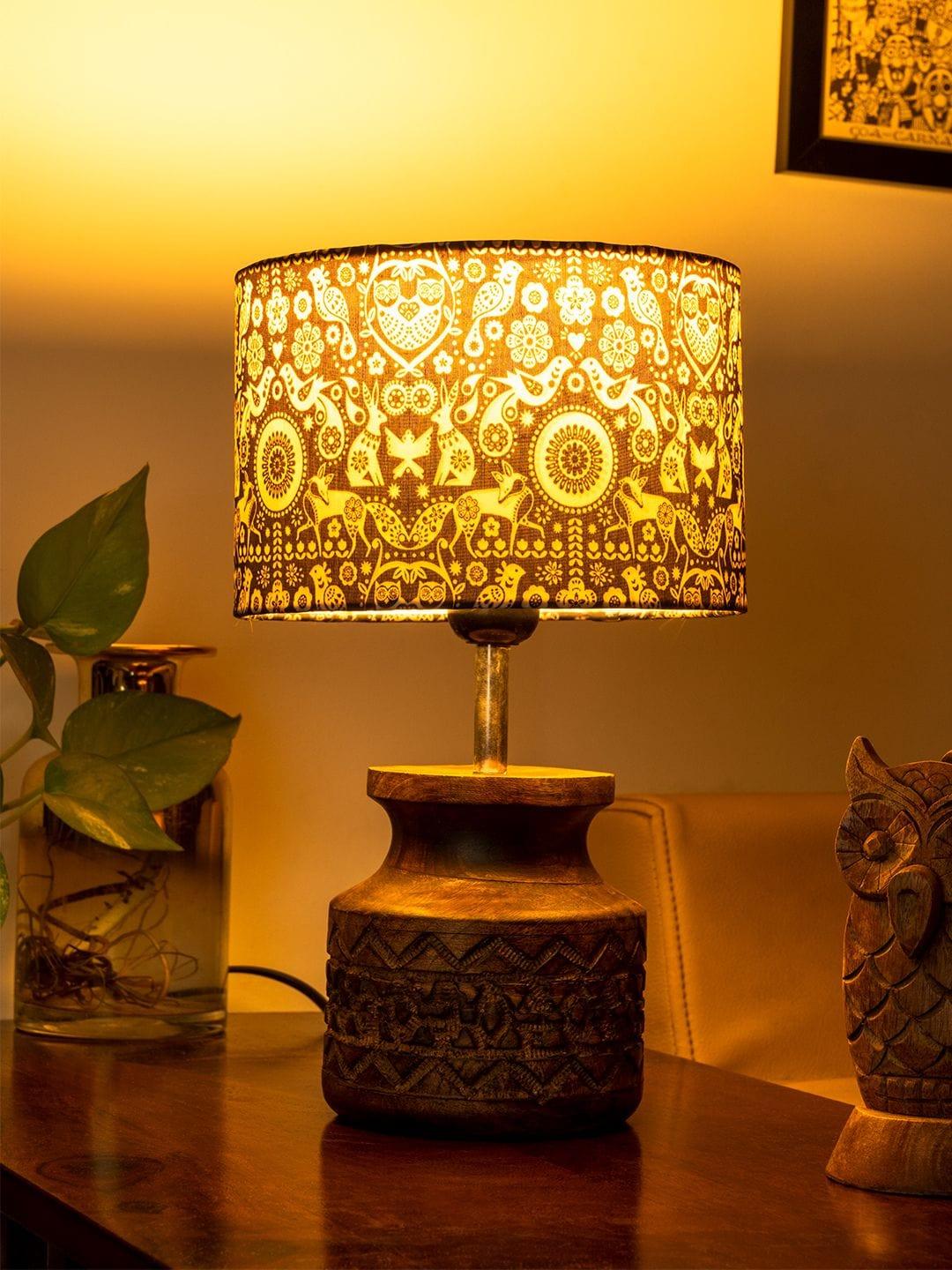The image captures a dimly lit room with the primary light source being an ornate lamp situated in the center. The lamp emits a warm yellow glow, casting soft shadows in the surrounding area. It features an intricate, cylindrical lampshade adorned with Pennsylvania Dutch-inspired designs, which include floral patterns and nature motifs such as birds, rabbits, foxes, and owls. The base of the lamp is carved from wood and showcases intricate engravings, resembling a snake-like design meandering across its surface. The lamp rests on a polished dark wooden table. To the left of the lamp is a lush green houseplant, housed in a jar with visible roots. To the right sits a carved wooden owl statue. Behind the lamp, a white wall forms the backdrop, with a small corner of an artwork visible at the top right corner. The bottom right corner reveals a piece of what appears to be a light brown or tan leather couch, suggesting the setting is a cozy, well-decorated home.